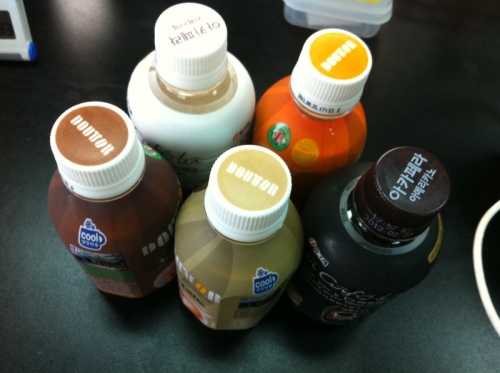This color photograph captures a collection of five plastic bottles, closely packed and centered in the frame, viewed from a bird’s eye perspective. Each bottle displays the logo "doto," indicating they are beverages from the Japanese coffee chain Doto. The bottles are a variety of colors – brown, white, orange, black, and caramel. Notably, the caps of the bottles, which are white, feature some Korean text on at least two of them, suggesting the drinks are Asian in origin. The image is well-lit from above, highlighting the glossy surface of the bottles. They are grouped together on a dark gray or black laminated countertop, with a couple of indistinct white objects visible around the periphery, enhancing the focus on the center arrangement. The close-up view and the lighting emphasize the contrast and the sleek design of the bottles, though the exact contents remain indistinguishable.